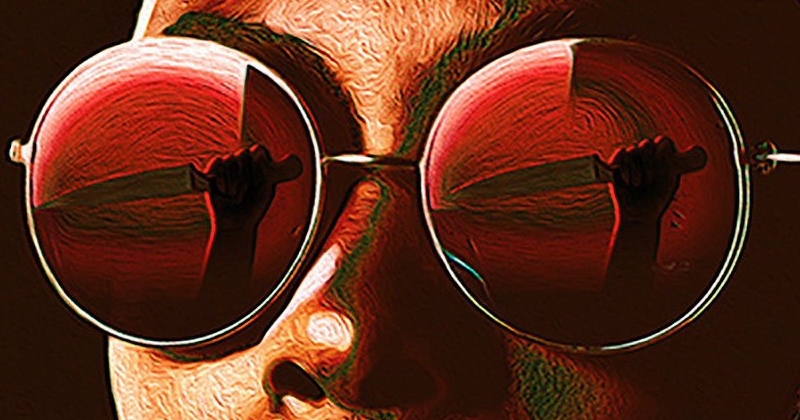This digital illustration, done in a pop art style, presents a partial close-up of a man's face, from the nose to the eyebrows. The artwork emphasizes high-contrast colors, with the skin shaded in a mix of orangey-tan and green hues. The man sports distinctive, round red sunglasses with silver rims, which dominate the image. Reflected in the mirrored lenses of the glasses is an eerie, repetitive scene: a silhouette of a hand gripping a large kitchen knife poised for action against a stark red background. The images in both lenses are identical, contributing to the unsettling and surreal atmosphere of the piece. The overall composition, flooded with red and green tones, lends a dark, dramatic twist to the visual narrative.